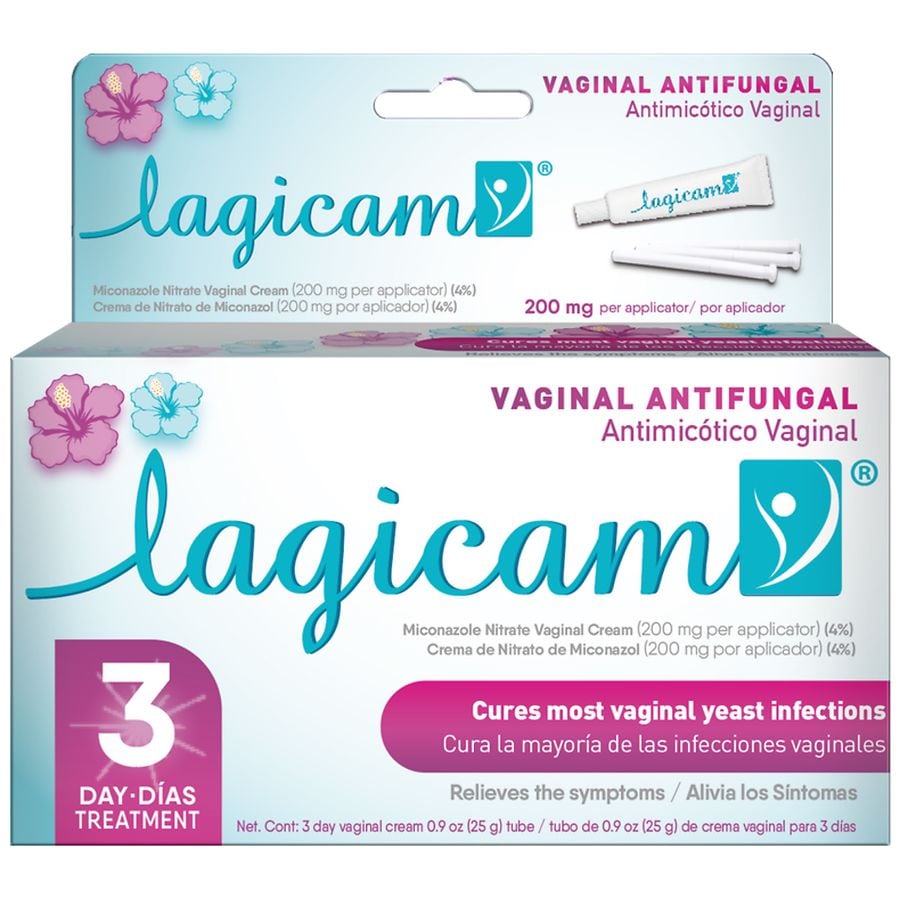The image displays the packaging for a vaginal antifungal cream called Lagicam. The box, measuring approximately six inches wide by two inches tall, features a light blue gradient background with the product’s name, "Lagicam," elegantly written in cursive turquoise text both at the top and bottom. The packaging includes a one and a half inch by four inch back hanger, facilitating easy display in a retail environment. Vibrant red and blue hibiscus flowers adorn the upper left-hand corners of both the hanger and the box, adding a touch of visual appeal.

In the lower left-hand corner, a pink-outlined banner reads "3-Day Dias Treatment" in white text, indicating the duration of the treatment. The upper right-hand corner of the box prominently displays the phrase "Vaginal Antifungal" in pink, followed by the ingredient details: "Miconazole Nitrate Vaginal Cream 200 milligrams per applicator," also provided in Spanish as "Crema de Nitrato de Miconazole.” Below this information, a red banner with white text assures users that the product "Cures Most Vaginal Yeast Infections," reiterating the same message in Spanish beneath it.

Additionally, there is an illustration of the cream tube and applicator on the packaging, providing a clear visual of the product inside. The design is cohesive, with blue and pink elements consistent across all sections, ensuring that all informational text is mirrored in Spanish, catering to a bilingual audience.